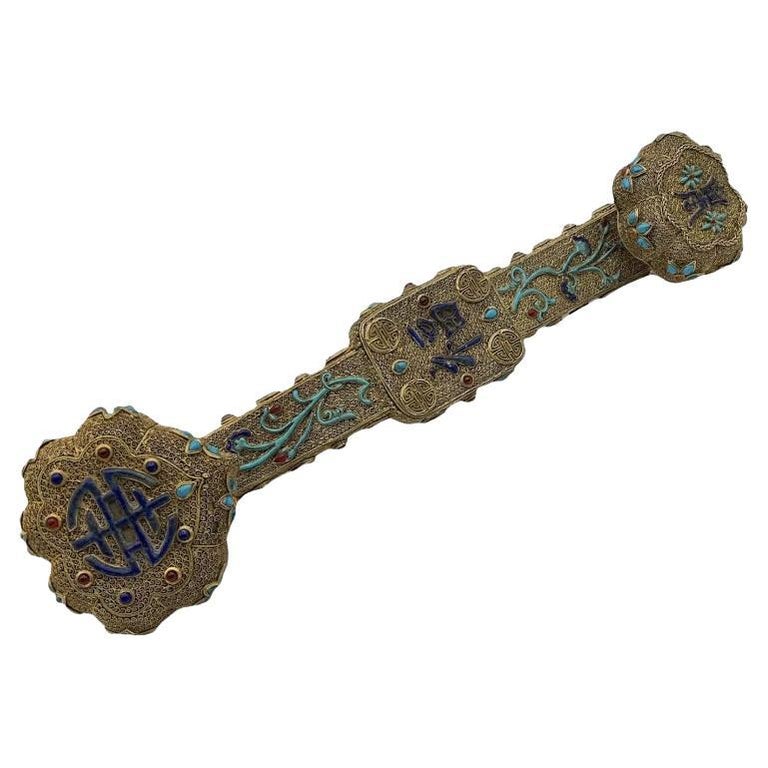The image features an ornate jewelry piece, primarily similar to a wristband, created from a gold or brass-colored fabric with a metallic sheen. The photograph, taken against a blank white background, highlights the intricate details of the piece. The jewelry is interwoven with a blue thread and embellished with turquoise, tear-shaped jewels that encircle the band. At one end, the piece terminates with two round balls connected by a thin, ruler-sized stick. The design includes several Asian characters on both ends and a central rectangular section. The left end showcases a heart-shaped insignia with additional blue detailing, while blue, red, and black beads fill the spaces throughout the piece. The right end features another distinct flower design in light and dark blue with red accents. Overall, the band displays antique qualities with its elaborate filigree and mixture of metal, fabric, chain-like elements, and multicolored gemstones.